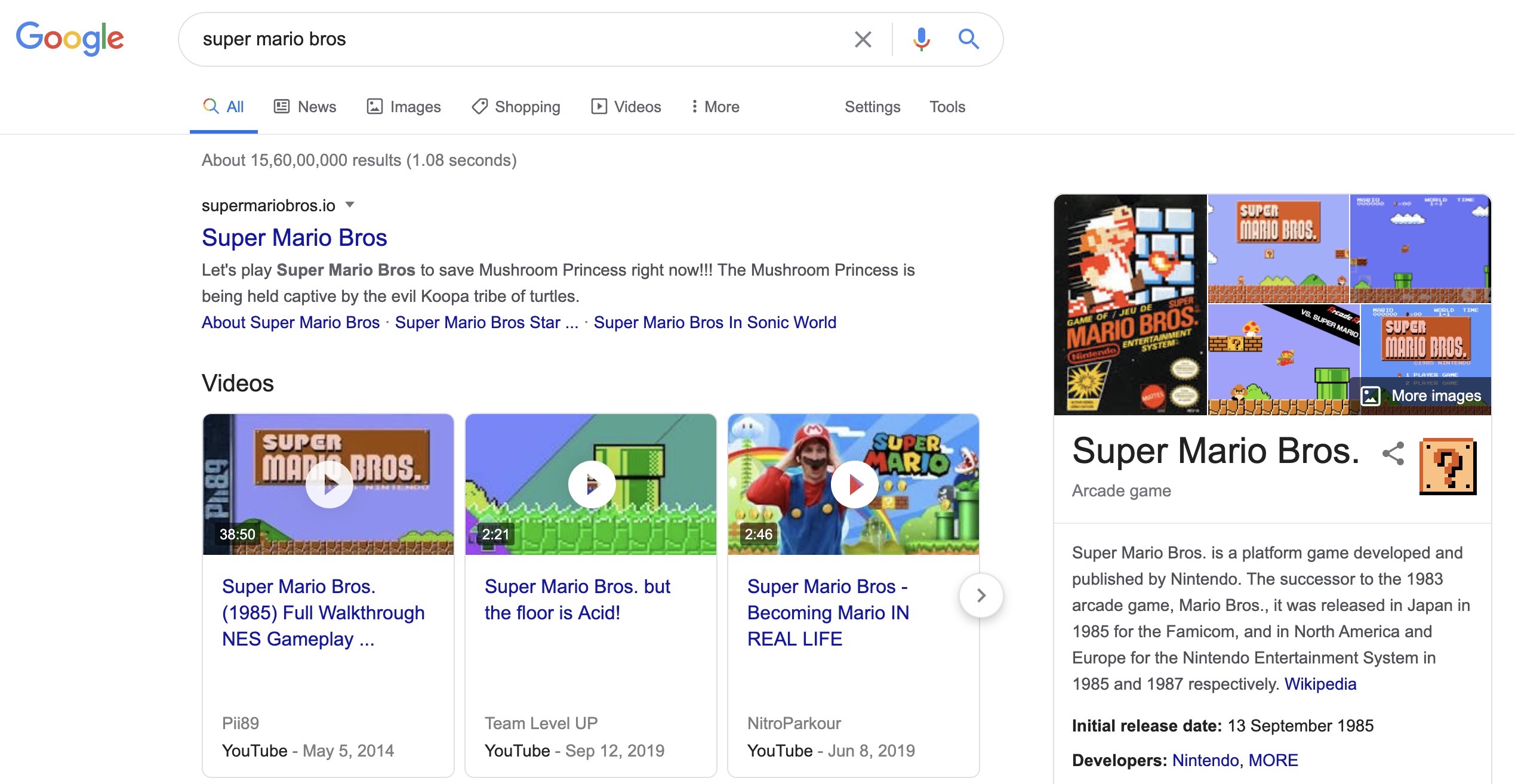The image depicts a Google search results page for "Super Mario Bros." The first result shown is for the website SuperMarioBros.io, followed by the official Super Mario Bros. website, which features the tagline "Let's play Super Mario Bros. to save Mushroom Princess right now." According to the site, the Mushroom Princess is being held captive by the evil Koopabra tribe of turtles.

Additionally, there is a section labeled "Videos" showcasing three different Super Mario-related videos you can watch on YouTube:

1. "Super Mario Bros. 1985 Full Walkthrough NES Gameplay"
2. "Super Mario Bros., but the Floor is Acid" posted by Team Level Up on September 12, 2019
3. "Super Mario Bros.: Becoming Mario in Real Life" posted by Nitro Parkour on June 8, 2019

The search options at the top of the page include categories such as All, News, Images, Shopping, Videos, More, Settings, and Tools, with "All" currently being featured. There is also a highlighted pop-up tile displaying the Super Mario Bros. game along with four images from it, labeled as an arcade game, accompanied by a brief description.